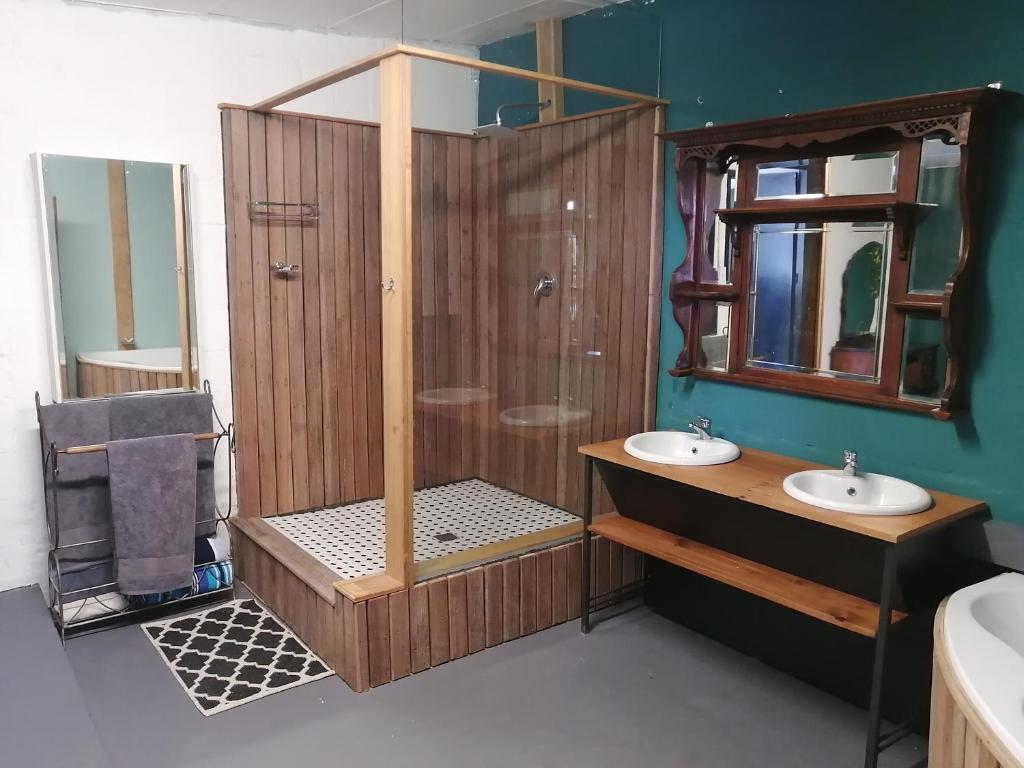The image depicts a minimalist bathroom featuring a striking contrast between its white left wall and a dark turquoise right wall. The room's floor is a flat grey concrete, adding to its simplicity. Dominating one side of the room is a spacious wooden shower, reminiscent of a sauna, with black and white tiling on the floor and a transparent plastic film on one side. In front of the shower lies a black and white crisscross patterned bath mat. Next to the shower, a freestanding towel rack with metal and wooden elements holds three grey towels.

Adjacent to this setup is a stylish wooden vanity with a metal frame and legs that support two plain white basins, each equipped with its own mixer faucet. Below the basins, a wooden shelf provides additional storage space. Above the vanity, an antique dark wood mirror vanity is attached to the wall, enhancing the bathroom's vintage charm. The vibrant teal blue-green wall behind the mirror and vanity adds a splash of color, unifying the room's eclectic yet cohesive design.